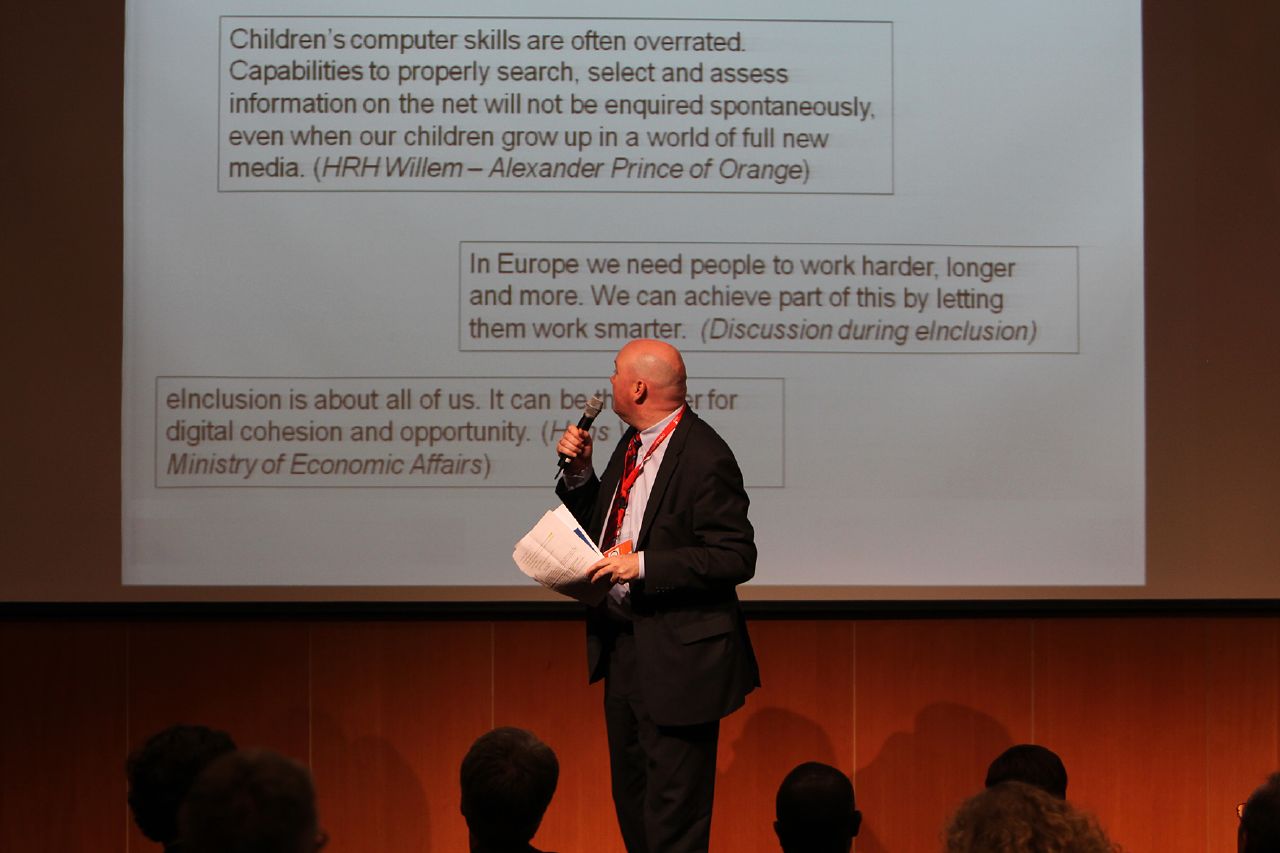In the darkened room, a white male presenter stands center stage, illuminated by the cool glow of a large projector screen behind him. Dressed in a black business suit with a white shirt and a red lanyard around his neck, he holds a microphone in his right hand and a stack of papers in his left. His balding head stands out against the dim environment. Facing slightly to the left, he gazes back at the projector screen to reference his talking points.

The screen features three text boxes stacked vertically. The top text box reads, "Children's computer skills are often overrated. Capabilities to properly search, select, and assess information on the net will not be acquired spontaneously, even when our children grow up in a world full of new media." It credits HRH Wilhelm, Alexander Prince of Orange. The middle text box emphasizes, "In Europe, we need people to work harder, longer, and more. We can achieve part of this by letting them work smarter. Discussion during inclusion." The bottom part of the screen mentions, "Inclusion is about all of us," referring to digital cohesion and opportunity before the text gets cut off.

The lower half of the audience is visible, with silhouettes and the backs of heads aglow in a warm, orange-red light. Scattered attendees hint at a sizeable audience witnessing the presentation, yet the focus remains sharply on the presenter and the crucial information displayed behind him.